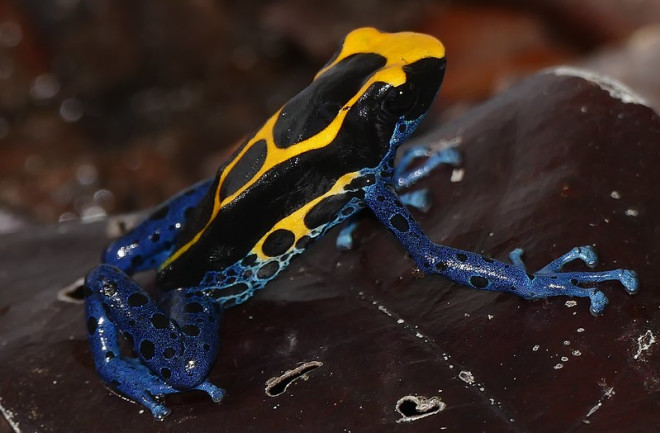This image captures a distinctive tree frog with a vibrant coloration and intricate patterns. The frog, slender and agile, displays a striking combination of blue on its legs and underbelly, adorned with black splotches. Its torso contrasts beautifully with yellow and black mottling, and its smooth, shiny skin accentuates these vivid hues. Perched atop a grayish-black surface, which could be a leaf or a rock, the frog grips it with long, delicate fingers. The background is artfully blurred, ensuring the focus remains solely on the frog and its perch. While the background hints at shades of orange, brown, black, gray, and white, these colors are obscured to maintain emphasis on the frog. Notably, the frog seems to have an extra foot, suggesting the possibility of an AI-generated image, adding a layer of intrigue to this already captivating subject.